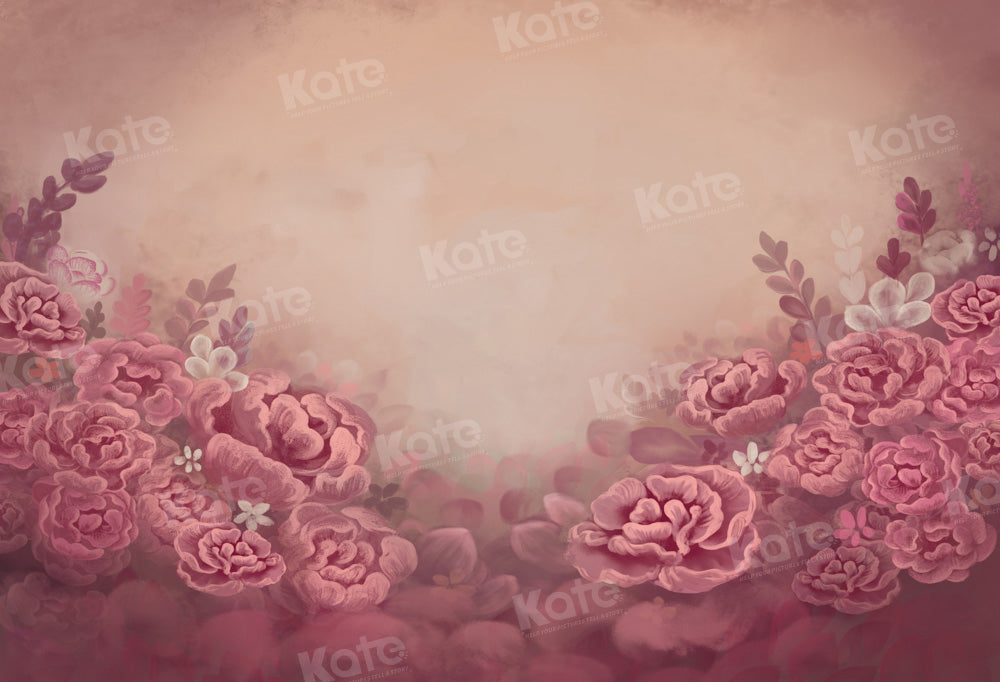This illustration is a vibrant stock image resembling a watercolor painting. It features layers of pink flowers with wrinkly petals, forming bowl-like and cabbage-like shapes that are likely peonies. The flowers are prominently positioned in an arc across the bottom and sides of the image, creating a lush, central focus. Between the flowers, hints of purple foliage can be seen, adding contrast and depth. The background is a foggy, creamy tan with off-white and slight gray hues, contributing to a misty atmosphere. A repeated watermark, reading "Keith Cabouquet" or "Kate," is visible across the entire image.